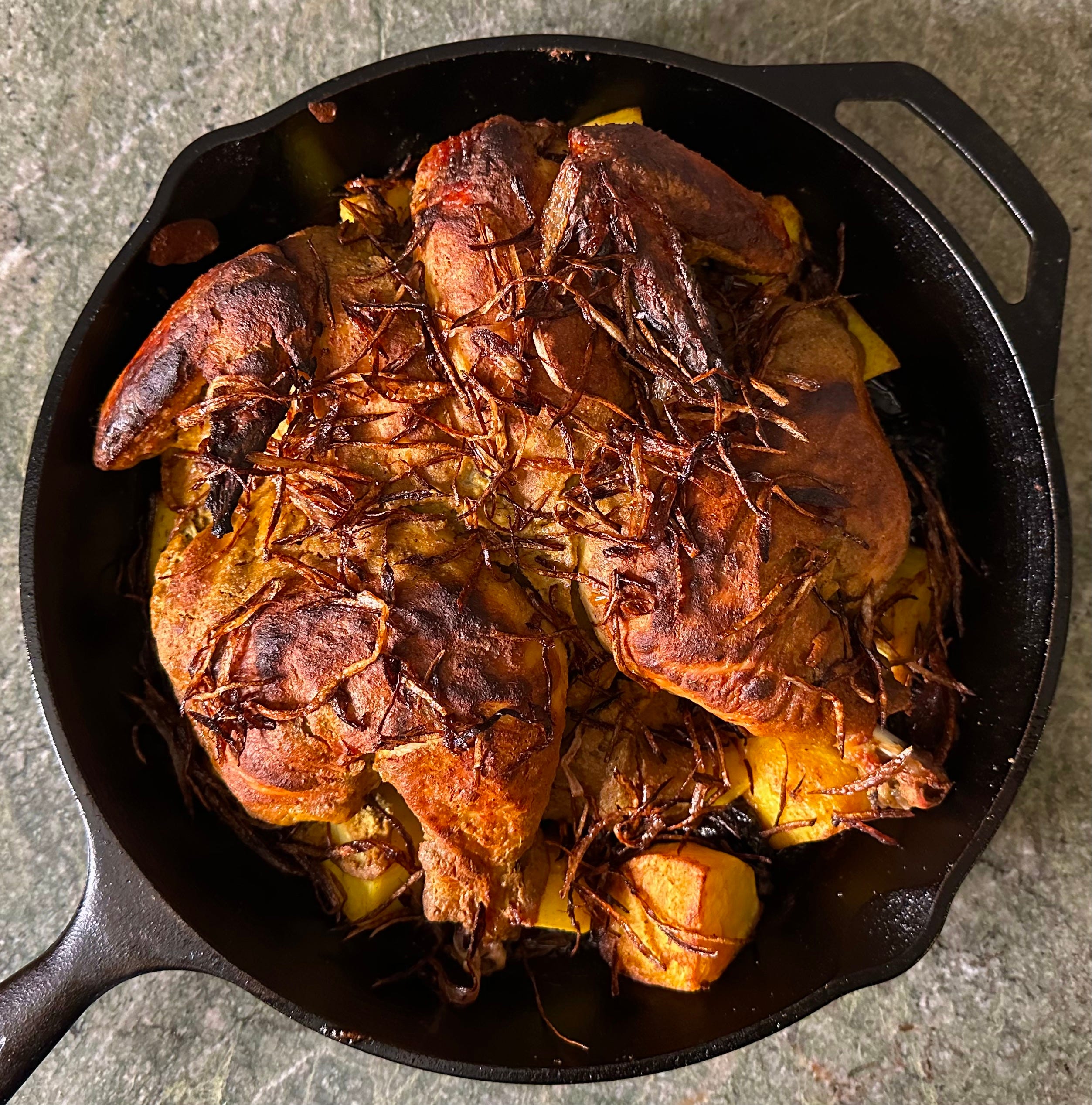This photo depicts a well-cooked, spatchcocked chicken nestled in a large cast iron skillet, which rests on a gray, stone-like countertop. The skillet features a handle on one side and a smaller handhold on the opposite. The chicken, browned to perfection with crisp, herb-laden skin, takes center stage, surrounded by golden, cubed potatoes. The potatoes, similarly caramelized and crispy, peek through beneath the chicken. A sprinkling of thinly cut, fried onions or herbs adds an additional layer of texture and flavor across both the meat and potatoes. The dominant colors in the scene are rich browns and golden yellows, contributing to an overall impression of a hearty, delicious meal, ready to be served.